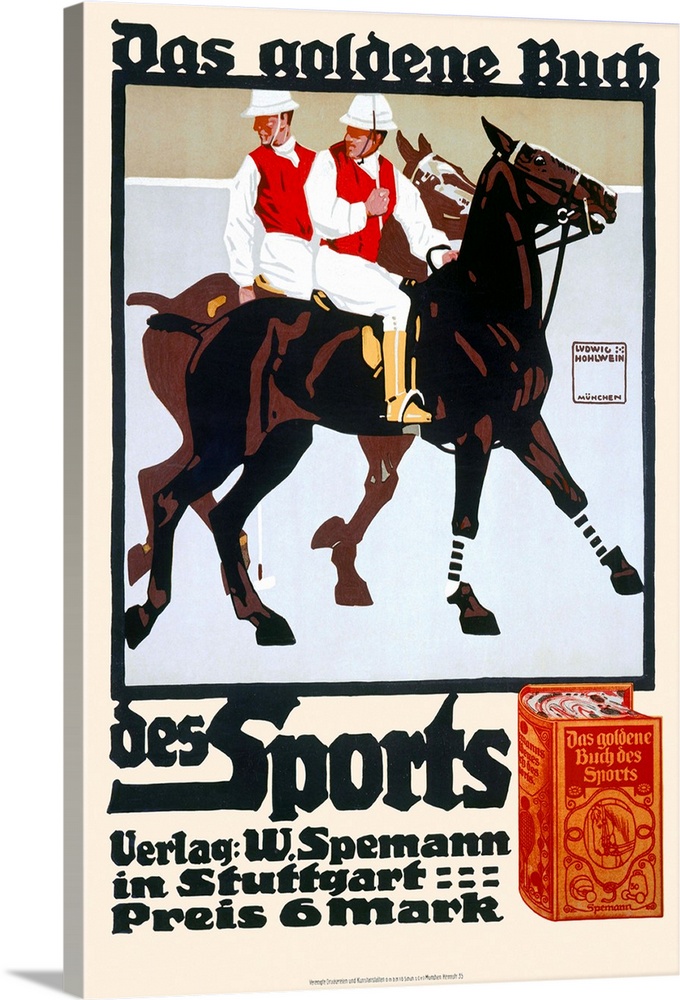The image depicts a 3D advertisement with a pink border set against a white background. The advertisement, which appears to be in German, prominently features the title at the top, reading "Das Goldene Buch," which translates to "The Golden Book." Beneath the title is a vintage-style illustration portraying two horse jockeys dressed in white uniforms complemented by red vests and hats, as well as yellow boots. They are riding brown horses, one dark and one light, both headed eastward. This scene seems to promote a horse-riding competition or game. Below the illustration, the text "Das Sports" is visible, followed by "Verlag W. Spiemann" and "Stuttgart." The entire advertisement has a slightly angled presentation, offering a visible side edge that adds to its 3D effect.